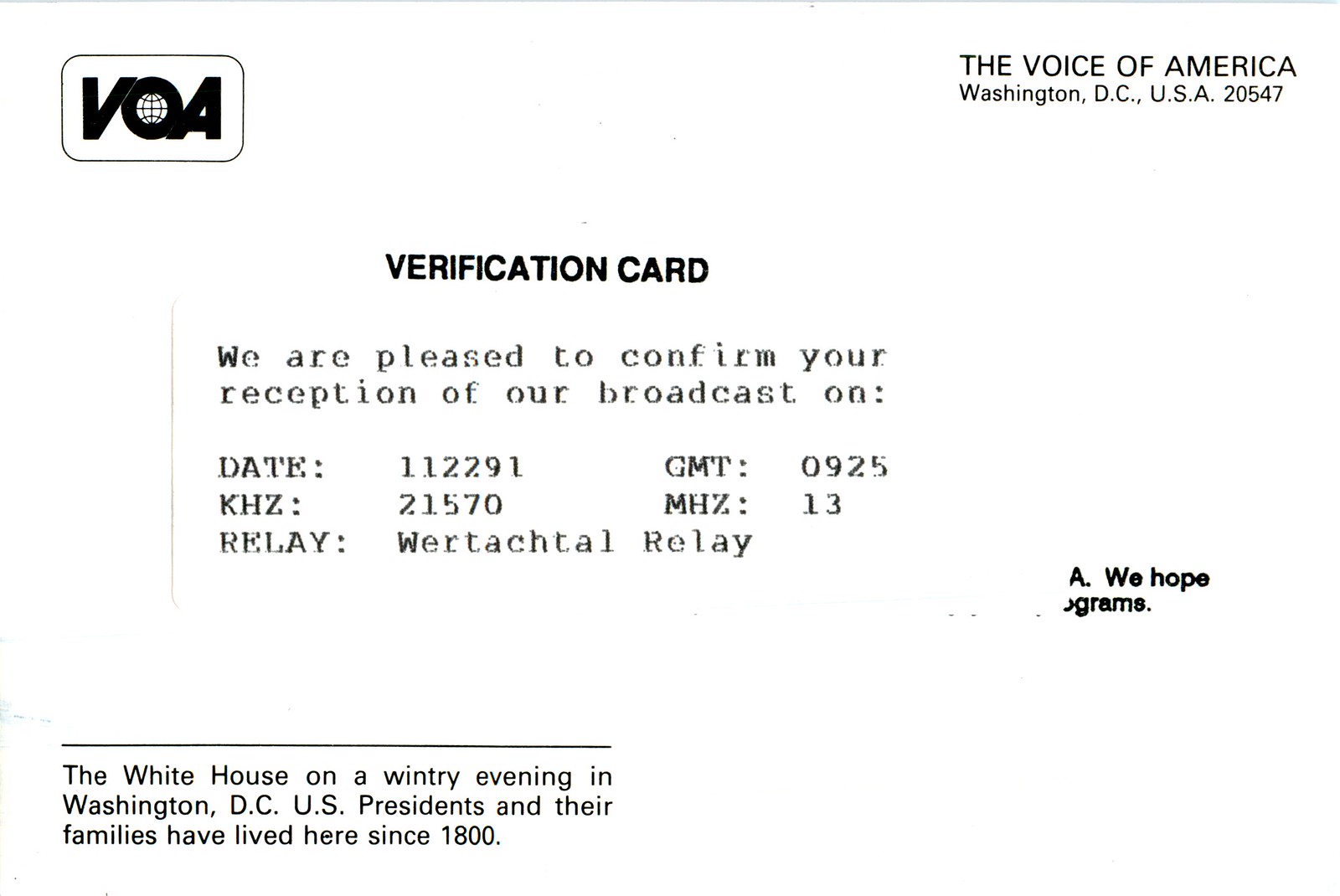The image displays a verification card for the Voice of America (VOA). The entire background of the card is white with multiple lines of black printed text. In the top left corner, there is a rectangle with a black border and a white interior containing the letters "VOA," where the "O" encircles a small world symbol. In the top right corner, the card reads: "The Voice of America, Washington DC, USA 20547." 

At the center of the image, the text "verification card" is prominently displayed in bold black letters. Following this, the card states: "We are pleased to confirm your reception of our broadcast on date: 112291, GMT: 0925, KHZ: 21570, MHZ: 13." Below this information, it includes a note: "Relay or tactile relay."

Toward the bottom of the card, there is additional text that reads: "The White House on a wintry evening in Washington DC. U.S. presidents and their families have lived here since 1800." Some lines and faded text might be present, suggesting age or wear.